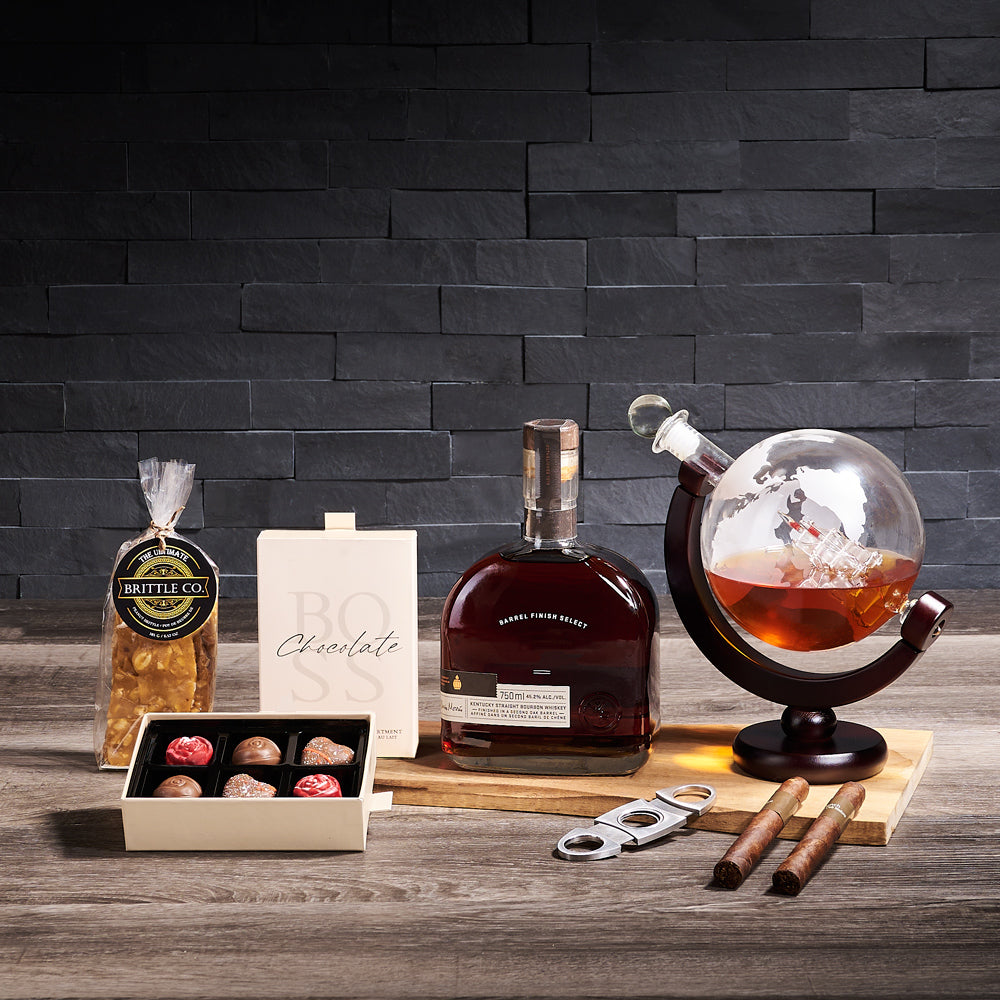The image features an array of products displayed on a brown wooden table. From left to right, the first item is a bag from The Ultimate Brittle Company, labeled "Peanut Brittle," filled with numerous pieces of brittle in a small, sealed bag. Next to it, there's a white box labeled "Chocolate," containing six chocolates—two red, two brown, and two drizzled with some type of coating. Following the chocolates is a bottle of Kentucky Straight Bourbon, labeled "Barrel Finished Select," with an alcohol volume of 45.2% and a capacity of 750 milliliters.

In the middle of the display, there's a glass globe-shaped decanter partially filled with brown liquid, likely whiskey, sitting on a dark brown horseshoe-shaped stand. In front of the decanter are two cigars accompanied by a cigar cutter. All these items rest on a cutting board against a backdrop of a black slate brick wall, creating a sophisticated and elegant presentation.